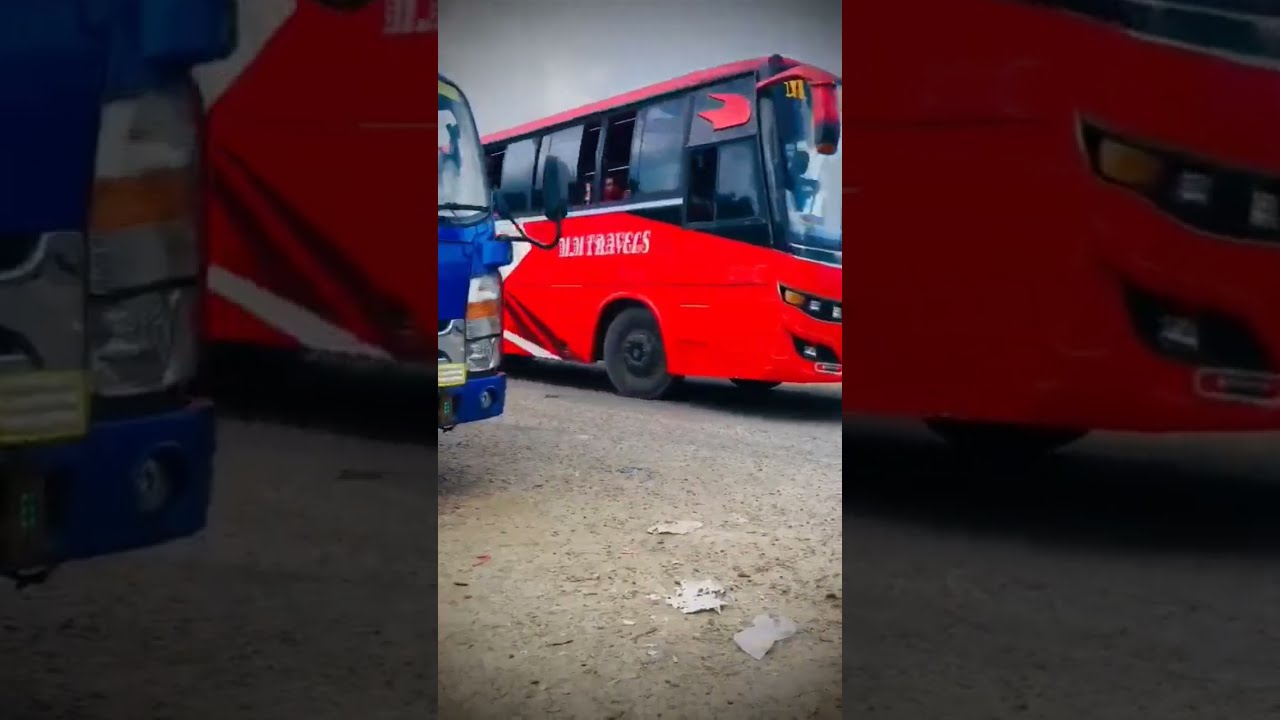The image is a digital photograph, captured from a screenshot of a social media video, depicting two buses parked on a flat, compacted dirt driveway. The photograph is composed of three sections: the central section showcasing the buses, and the left and right sections zoomed in on parts of the central image, with black filters added to indicate the original picture's insufficient size for the screen.

In the center section, on the left side is a blue bus, partially visible, with just the right side of its headlights and a bit of its front bumper showing. To the right is a red bus with large, black windows, most of which are slid open. The front of the red bus faces right, exposing shiny, black-rimmed rubber tires and a partially blurred marking that may be a number or text in a different language.

The left zoomed-in section focuses on the front bumper of the blue bus and a part of the red bus's side, including the compacted dirt road. The right zoomed-in section highlights the front bumper of the red bus and more of the dirt road. Notably, one of the windows of the red bus is open, revealing a person's head behind it. The ground is strewn with gray-colored leaves, and the sky is a dull, dark gray, contributing to the overall muted color palette of red, black, white, blue, and brown.